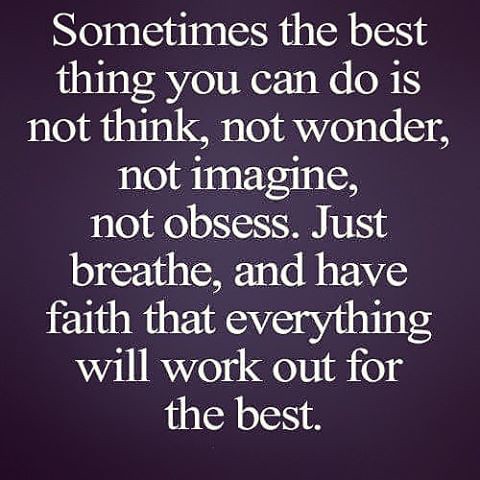The image features an inspirational quote graphic commonly found on social media platforms like Facebook or Instagram. The background is a gradient that transitions from dark purple to dark gray, with a lighter hue towards the center that darkens radiantly towards the edges. There are nine lines of centered white text that read: "Sometimes the best thing you can do is not think, not wonder, not imagine, not obsess. Just breathe and have faith that everything will work out for the best." The minimalist design emphasizes the motivational message, with the text standing out against the solid, dark gradient background.